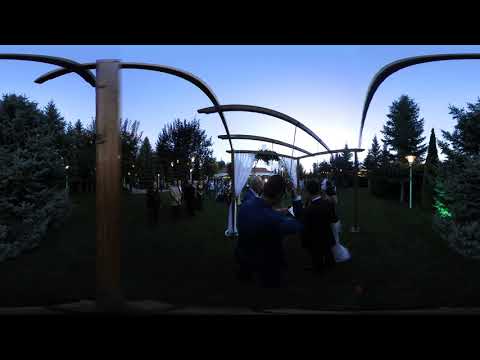The photograph captures an outdoor wedding ceremony set against a backdrop of clear blue skies and lush natural greenery. Central to the image are several photographers, whose presence slightly obstructs the view of the bride and groom. The ceremony is framed by an archway, under which the couple presumably stands. Guests, attired in elegant dresses and suits, are seated and standing in the background. The setting sun casts a diminishing light, enhancing the evening ambiance. The scene is enclosed by trees and a wooden pole on the left side, with a solid black border framing the top and bottom of the image, conveying a sense of a serene, well-attended event at dusk. The overall palette includes shades of green, blue, white, tan, and black.